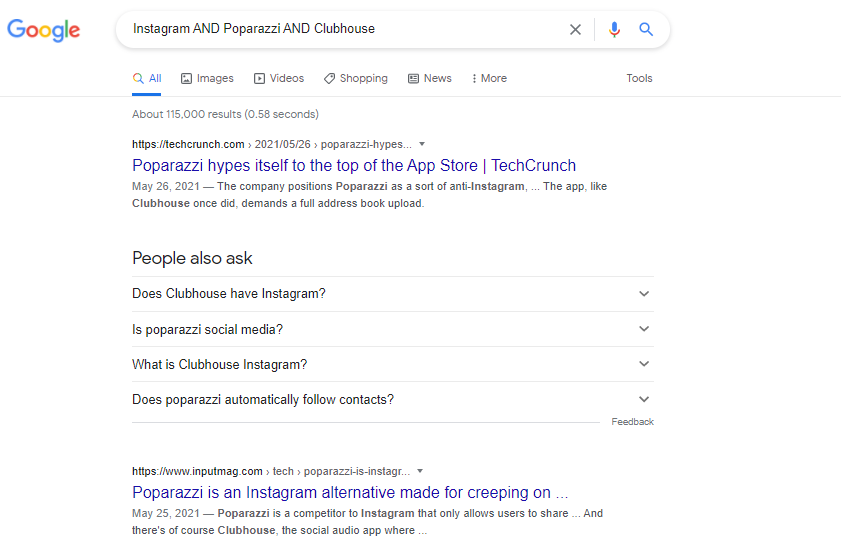A detailed screenshot captures the results of a Google search page, primarily focused on various social media platforms and applications. The search page features a diverse array of options including "All," "Images," "Videos," "Shopping," "News," and "More." The search yielded approximately 115,000 results in a rapid 0.58 seconds.

Prominently displayed at the top are sponsored links and trending articles. Highlights include discussions surrounding applications like Paparazzi, Instagram, and Clubhouse. A multitude of search snippets and URLs point to sources such as https://crunch.com, with an article from 2021, and https://www.inputmag.com, emphasizing the coverage of these platforms.

One notable snippet details the prominence of the Paparazzi app on the App Store and its comparison to Instagram, citing privacy concerns and the unique demand for full address book uploads by Clubhouse. Questions such as "Does Clubhouse have Instagram?" and "Is Paparazzi a social media platform?" hint at the curiosity among users about the functionalities and privacy implications of these apps.

The background of the screenshot is white, providing a clean and uncluttered visual that focuses the viewer’s attention on the search results and information presented.